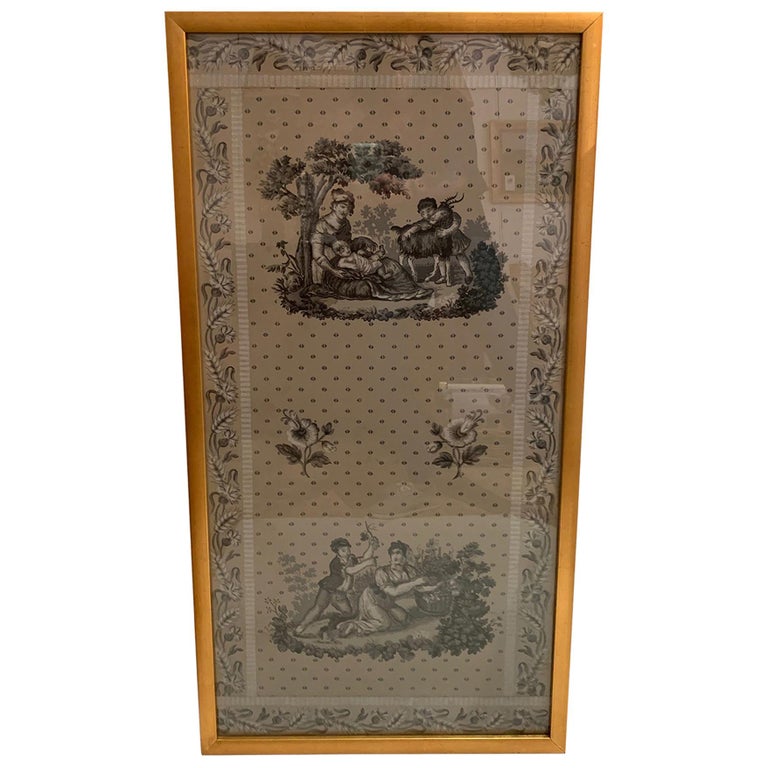The image portrays a vertically framed piece of art in a simple, rectangular wooden frame with a medium oak coloring. The artwork inside the frame appears to be a tapestry with a light tan or beige background. The border of the tapestry is intricately embroidered or adorned with leaves and flowers, possibly cattails and small daisies, running along the top, sides, and bottom edges. The art within the frame is divided into two distinct scenes.

In the upper section, a serene outdoor scene unfolds under a sparse tree with the leafiest branch extending over a small group of people. Seated beneath the tree is a woman cradling an infant, next to whom stands a young boy embracing a horned animal, likely a goat. This scene is flanked by two embroidered flowers in the center.

The lower section of the tapestry depicts a woman kneeling on the ground, possibly engaging with a planter or basket. Behind her is a child, seemingly holding an object that could be a twig or perhaps something else. This segment also includes embellishments of flowers, adding to the rustic charm of the piece. The colors used in the artwork are predominantly darker grays, greens, and various shades of beige, giving the entire piece a somewhat monochromatic and antique appearance.